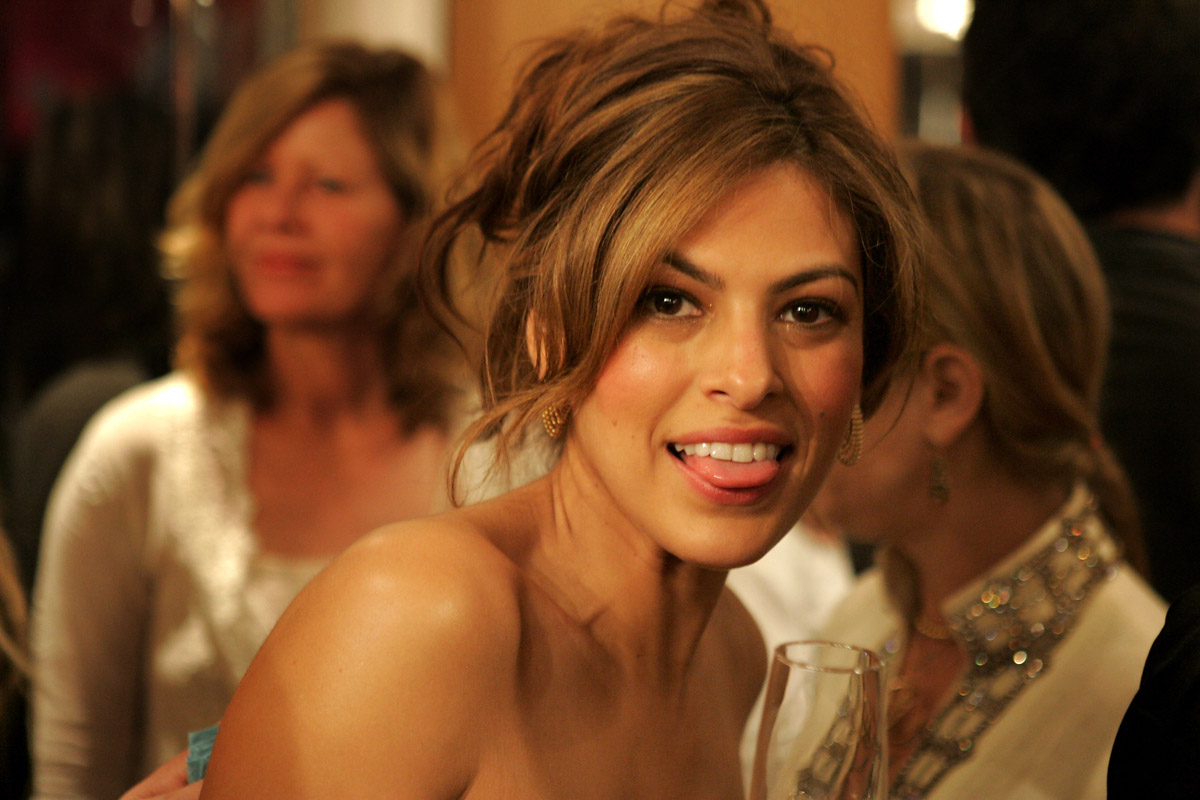In the image, the focus is on a woman positioned at the center, sticking her tongue out directly towards the camera. The background, though blurred, suggests an indoor setting with visible walls and light fixtures, indicating an evening formal event. A few people are discernible in the background, adding to the ambiance. The color palette includes shades of tan, pink, red, black, white, silver, and gray, creating a dynamic yet harmonious balance. The overall atmosphere is lively and sophisticated, enhanced by the woman’s playful expression against the formal backdrop.